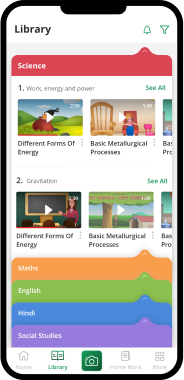A detailed caption for the image:

"The image showcases a vibrant and colorful screenshot of an educational app open on an iPhone. The clarity of the photo reveals a well-lit screen, though the text appears slightly blurred. In the top left corner, the words 'Real Library' are inscribed in black text. Adjacent to this, on the right-hand side, are two icons: a green bell for notifications and a green funnel icon, likely for filtering. 

Dominating the screen is a prominently displayed tab labeled 'Science' in white text set against a red background. Beneath this tab, a section titled 'Work, Energy, and Power' is marked as number one, with a 'See All' option on its right. Below this heading, two video thumbnails are clearly visible. The first thumbnail is labeled 'Different Forms of Energy' and appears to be from an animated video. The second thumbnail bears the title 'Basic Metallurgical Processes,' also featuring an animation. A third thumbnail is partially visible, indicating another animated video whose title is cut off.

The second section is titled 'Gravitation' and listed as number two. The animations here follow a similar pattern, with the first video again showing 'Different Forms of Energy' and the second being 'Basic Metallurgical Processes.' A third animated video is partially hidden from view.

Lower on the screen, there are several colorful tabs, though these are not expanded. They include 'MADS' in an orange tab, 'English' on a lime green background, 'Hindi' on a blue background, and 'Social Studies' in a purple tab.

At the very bottom of the screen are the typical navigation icons of the app. From left to right, they include a 'Home' icon, a 'Library' icon represented by a book, a central camera button, a 'Homework' icon depicted as a notepad, and a 'More' option illustrated by four squares arranged in a grid."